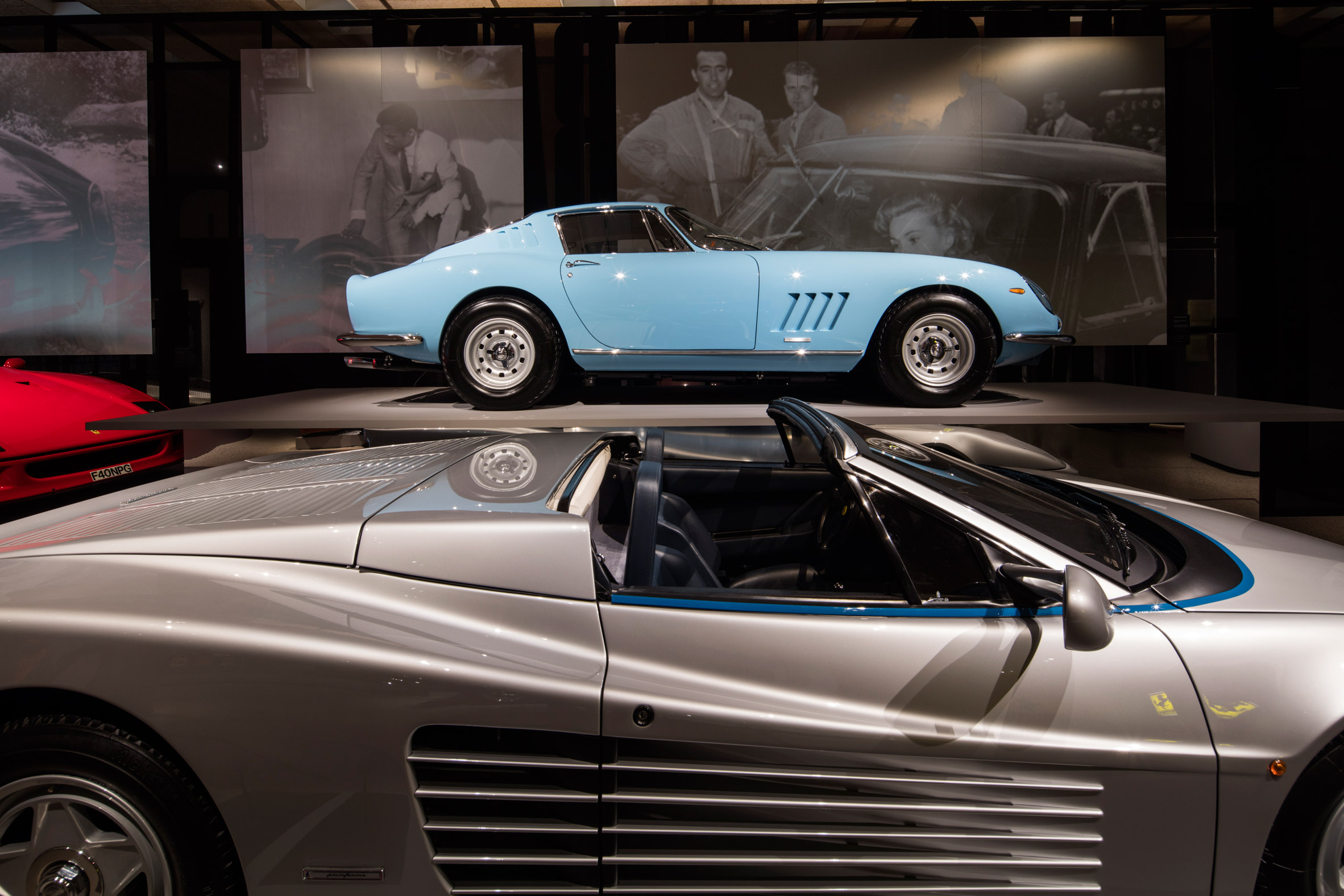This image, likely taken in a car museum, showcases a sleek automotive display with a focus on sporty, modern designs. In the foreground, the centerpiece is a compact, silver sports car convertible with a futuristic aesthetic. It features a blue trim accentuating the door and front, adding to its dynamic appearance. The two-seater vehicle boasts black interior and striking rim detailing, exuding a sense of speed and agility.

Positioned behind it is a stylish powder blue sports car, also a two-seater. This vehicle carries elements reminiscent of classic American muscle cars, complemented by silver rims and black wheels, blending vintage charm with contemporary lines. 

The backdrop includes black and white photos, seemingly from the 1950s, depicting racers and men in tuxedos, adding a nostalgic touch to the modern display. Off to the back left, the front of a red sports car is visible, teasing the presence of yet another high-performance vehicle. The overall scene is set against a predominantly dark background, which highlights the featured cars and the historical imagery.